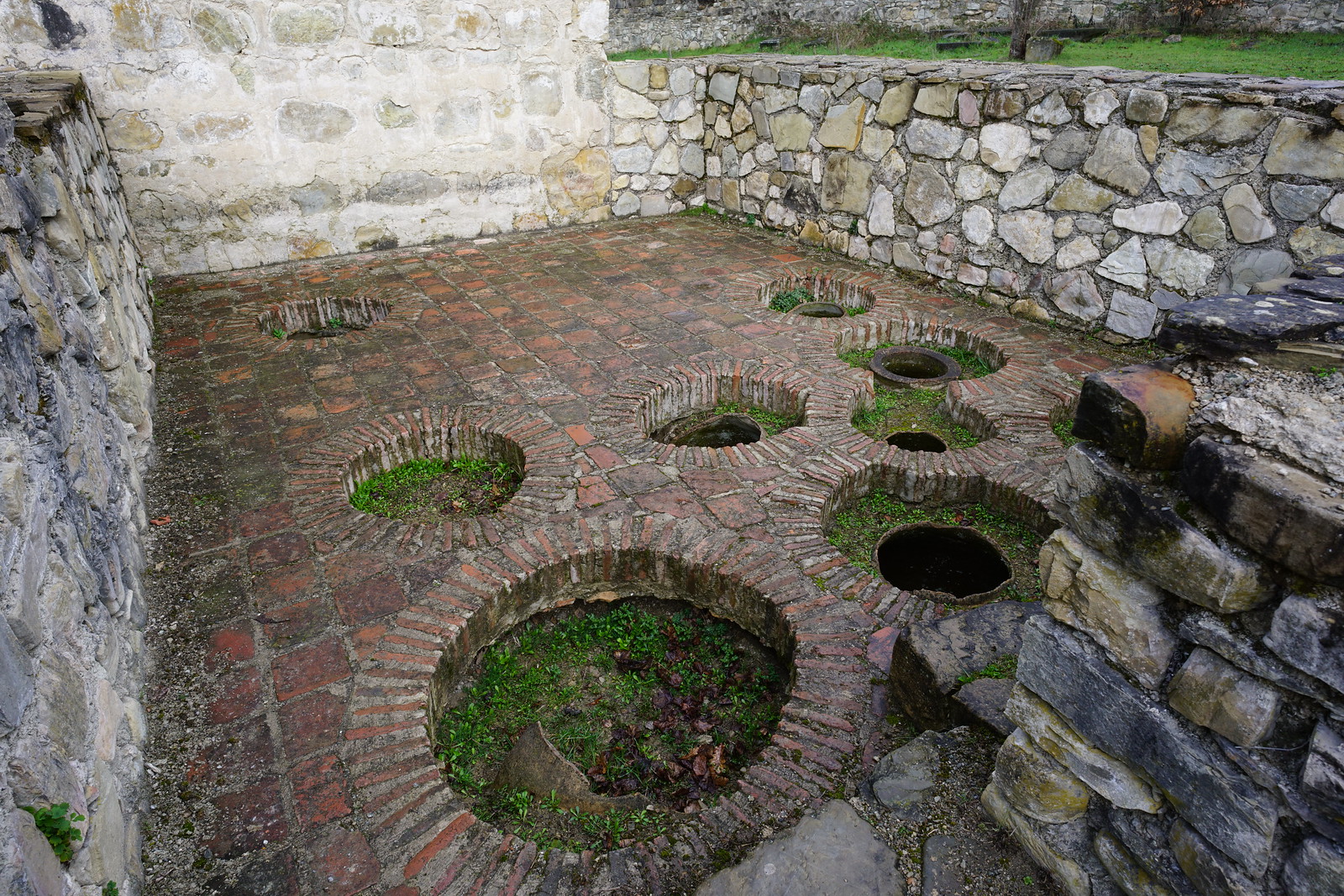This vivid image, captured in color and in landscape format, showcases a fascinating archaeological site set outdoors. Dominated by a meticulously constructed stone wall, which stands at least three feet tall and serves to retain the elevated ground, the site appears to be the remnants of an ancient building's foundation. The primary area within the stone walls is a floor section composed of neatly arranged brick tiles. Intriguingly, the brick floor features a series of precisely cut, large circular holes, each filled with green grass and specks of moss and fungus, hinting at nature reclaiming this once-structured space. These round cavities might have been part of the old plumbing system or designed as planting pockets, possibly intended for a pond or fountain that is now devoid of water. The attention to detail in the stonework and brickwork suggests a significant amount of effort and craftsmanship went into the original construction, even as the site now shows signs of disrepair and exposure to the elements.